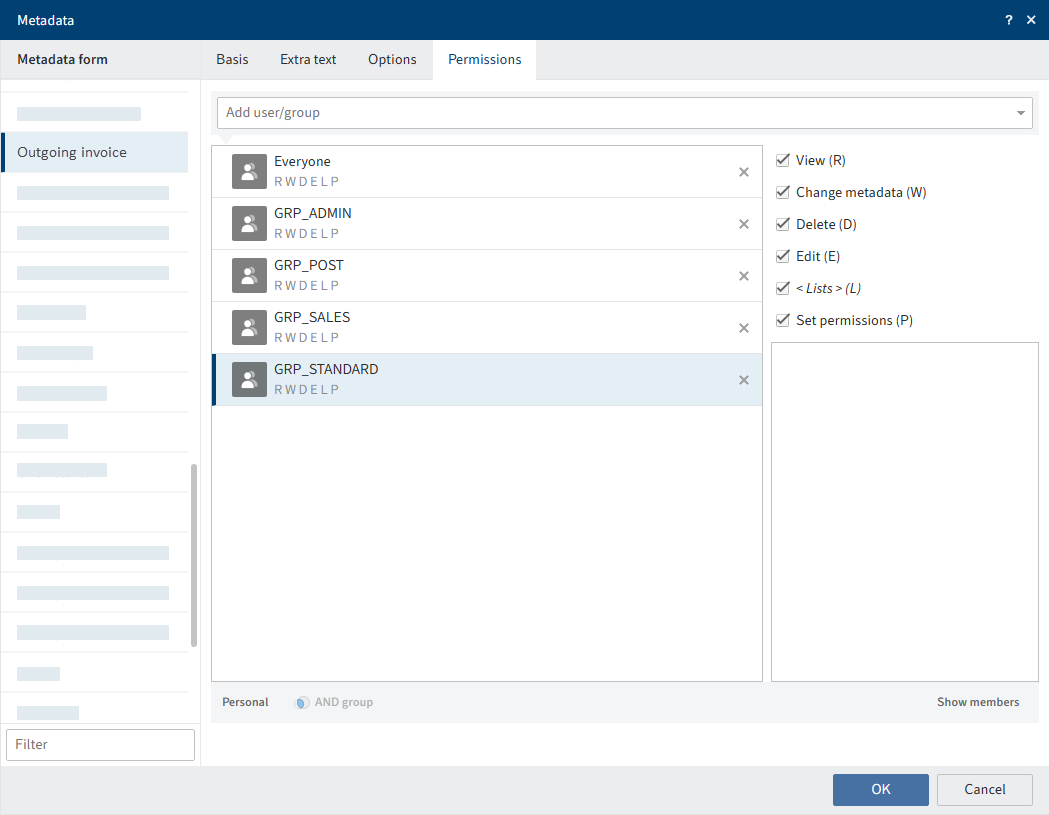This image is a screenshot from a laptop, displaying a detailed interface focused on metadata and permissions management. At the top of the interface, a long blue header stretches from the upper left-hand corner to the upper right-hand corner. The header's upper left reads "Metadata," while the upper right has a question mark icon followed by an 'X'.

Below this, a secondary row features a series of tabs labeled: "Metadata Form," "Basis," "Extra Text," "Options," and "Permissions," with "Permissions" highlighted in white and its font rendered in blue, indicating the active tab. The rest of the tabs in this row are in light gray.

The main body of the interface is divided into two primary columns of information. The left column, although partially obscured, lists various rows. The only visible row reads "Outgoing Invoice," marked by a thin blue stripe to its left. At the bottom of this column, there is a box labeled "Filter."

The right column begins with a header row labeled "Add User/Group." Below this, it divides into two sub-columns. The left sub-column lists five rows: "Everyone," "GRP Admin," "GRP Post," "GRP Sales," and "GRP Standard," with "GRP Standard" highlighted in light blue, signifying its selection. The other entries have a white background.

The right sub-column features a series of checkboxes labeled: "View," "Change Metadata," "Delete," "Edit," "List," and "Set Permission," all of which are checked off. Finally, at the bottom right of the interface, there are two buttons: "OK" (highlighted in blue) and "Cancel."